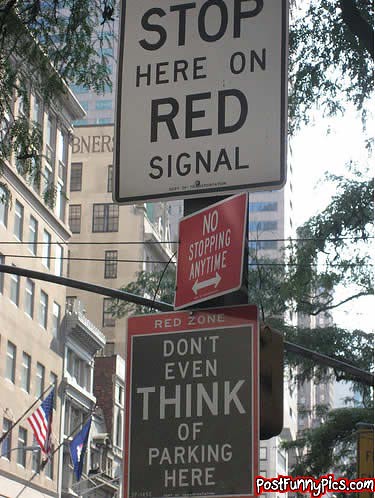The image displays a series of street signs, each with its own distinct design and message. At the top, there is a white square sign with the text "STOP HERE ON RED SIGNAL" in bold black letters. Directly beneath it, there is a smaller red and white square sign with white lettering that reads "NO STOPPING ANY TIME," accompanied by a double-headed arrow pointing in both directions. Below this, a slightly larger square sign features a prominent red border and header, with the main text "DON'T EVEN THINK OF PARKING HERE" in stark white letters against a black background. In the lower right-hand corner of this sign, a small print directs viewers to the website "postfunnypics.com" for additional content. The background behind these signs shows a bustling urban street with various buildings and a hint of greenery, adding context to the setting.